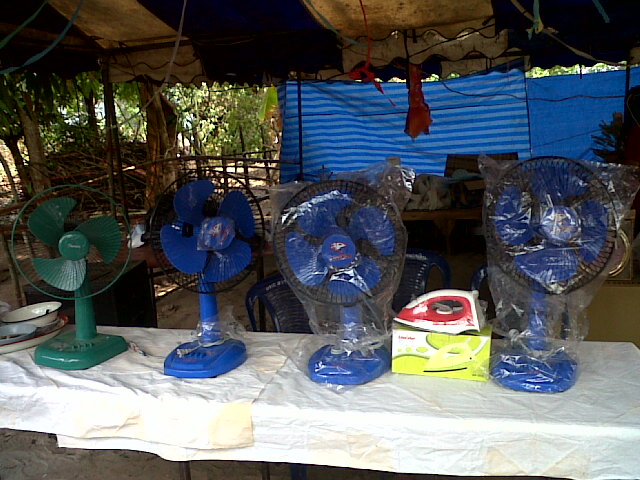This photograph captures a scene set under a tent-like structure with various fabrics creating a makeshift roof. In the foreground, there's a table draped with a white cloth, upon which four tabletop electric fans are neatly arranged side by side. The fan on the far left is distinctively dark green with a matching green housing that encloses the blades. The remaining three fans are dark blue, with plastic wrapping around two of them, and their black housings either removed or missing. Among these blue fans, an iron in its box is placed between the two on the right. The iron, sporting a red and white color scheme, faces the camera with its top side visible. In the background, blue tarps hang down, indicating a temporary setup, and additional items are scattered across a secondary table. The setup is surrounded by trees, with blue round metal chairs and various cookware items such as bowls on a plate, adding to the eclectic scene.